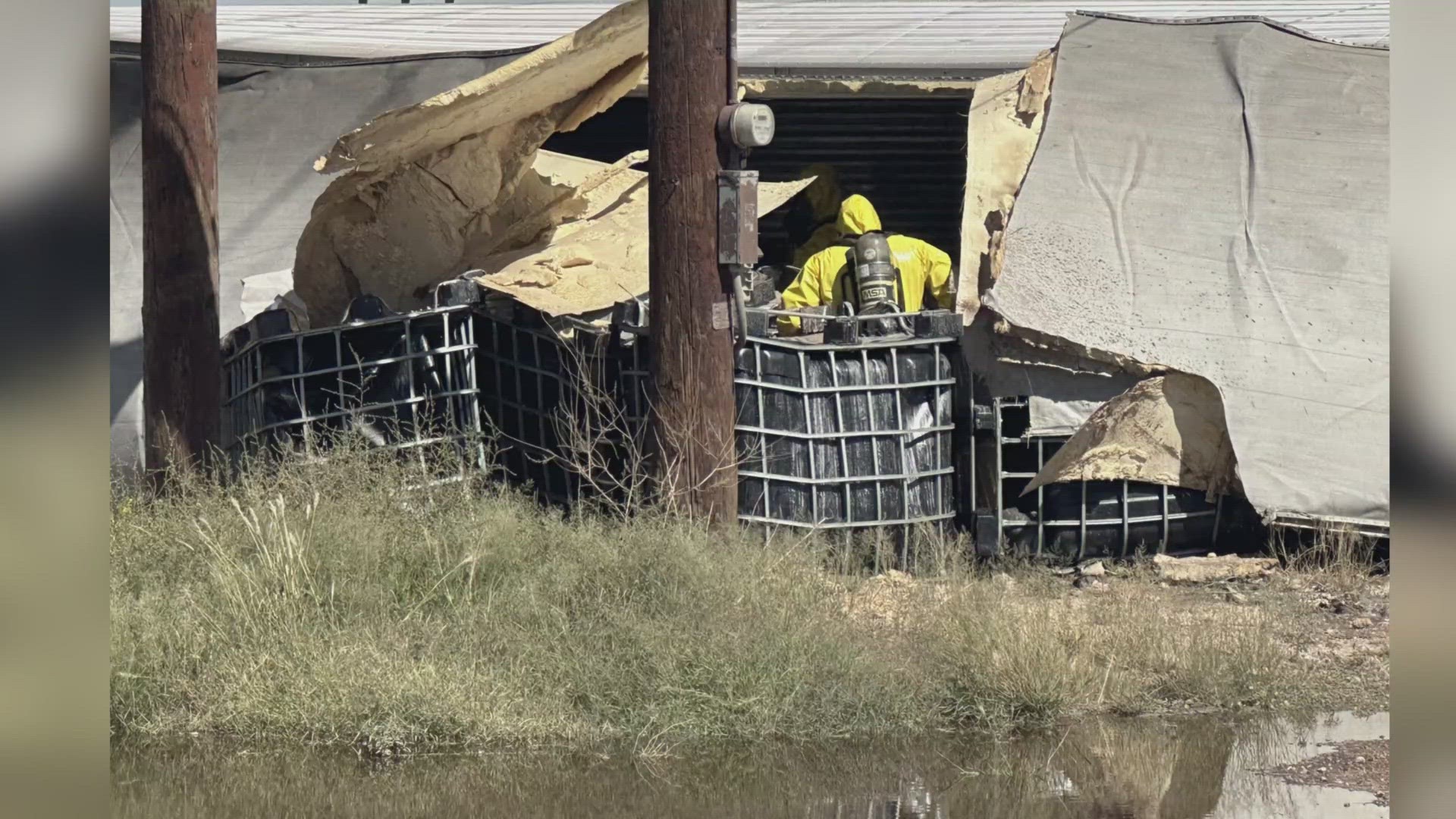The daytime photograph captures an outdoor scene centered around a dilapidated building with a gray roof. The structure appears heavily damaged, adding to the sense of decay in the environment. A person wearing a yellow hazmat suit and carrying a mask and an oxygen tank on their back is approaching the entrance, visible from the waist up. Surrounding the person is a terrain consisting of muddy, dirty patches with dead and tall grass intermingled. Scattered around the area is trash and garbage, contributing to the scene's disarray.

Noteworthy elements include a grid-style metal fence that runs alongside the scene, creating a boundary. The bottom portion of the image shows a small puddle or possibly a section of a stream, adding a reflective quality to the ground. On the far right, there's gray cardboard set up as a makeshift barrier. In the background, two large utility poles—likely power poles—tower over the area, enhancing the image's sense of isolation and abandonment. The overall clarity of the photo is vivid, taken under clear daylight conditions, which highlights the desolate and disordered state of the surroundings.